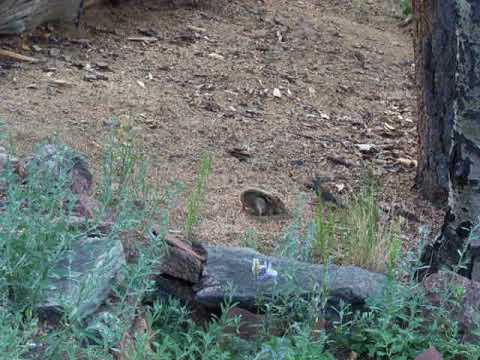This is an outdoor photograph taken during the daytime, measuring approximately four inches wide by three inches tall, showcasing a natural scene filled with elements of a forest floor. At the bottom of the square image, tall blades of green grass and weeds, speckled with a bit of brown, rise up among large, stacked gray and brown rocks forming a rough barrier. Some stems even show buds of white and blue flowers.

In the middle portion of the photo, extending to the upper part, the ground transitions into a slanted hillside covered with brown dried dirt, dotted with small rocks, wood chips, and fallen leaves. Among this dried foliage, there are scattered pine needles and pine cones adding texture to the landscape.

Dominating the central focus is a small tan chipmunk, distinguishable by the black and white stripes running along its back. The chipmunk's short tail is curved upwards, pointing towards the sky. It appears to be engaged in foraging, its face down in the ground, likely searching for nuts. Adjacent to the chipmunk, on the right side and extending from bottom to top, stands the base of a tree trunk, while in the upper left corner, a fallen tree trunk lays across the view.

This detailed outdoor scene captures both the tranquil, rugged beauty of a forest floor and the small woodland creatures that inhabit it.